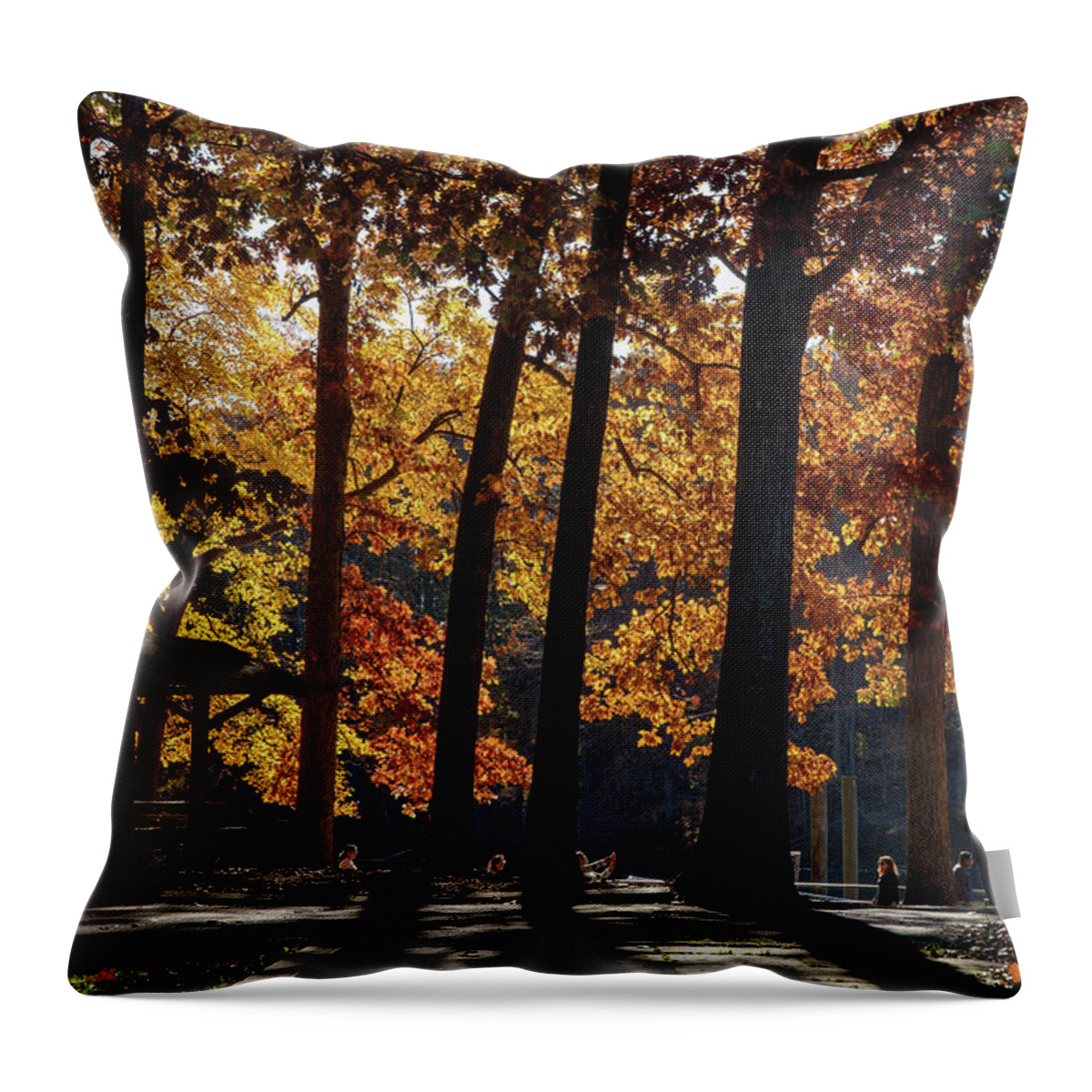The product listing image features a throw pillow against a plain white background with faint shadowing underneath. The pillow showcases a high-resolution photograph of an autumn scene in a park, printed across its surface. Dominating the image are tall trees with yellow, brown, and orange leaves, signifying the season's change. The trees' thick branches create a dense, shadowed canopy that extends off the edges of the pillow. At the bottom of the picture, the bases of the trees are visible, rooted in a grassy area with some possible flowers in the bottom right corner. Scattered among the trees, some people can be seen enjoying the park—sitting on the grass, standing near the trees, and walking along a sidewalk. In the distance, hints of a structure and what might be a body of water or lake add depth to the scene. The shadows cast by the trees contribute to the image's overall dark and enchanting autumnal atmosphere.